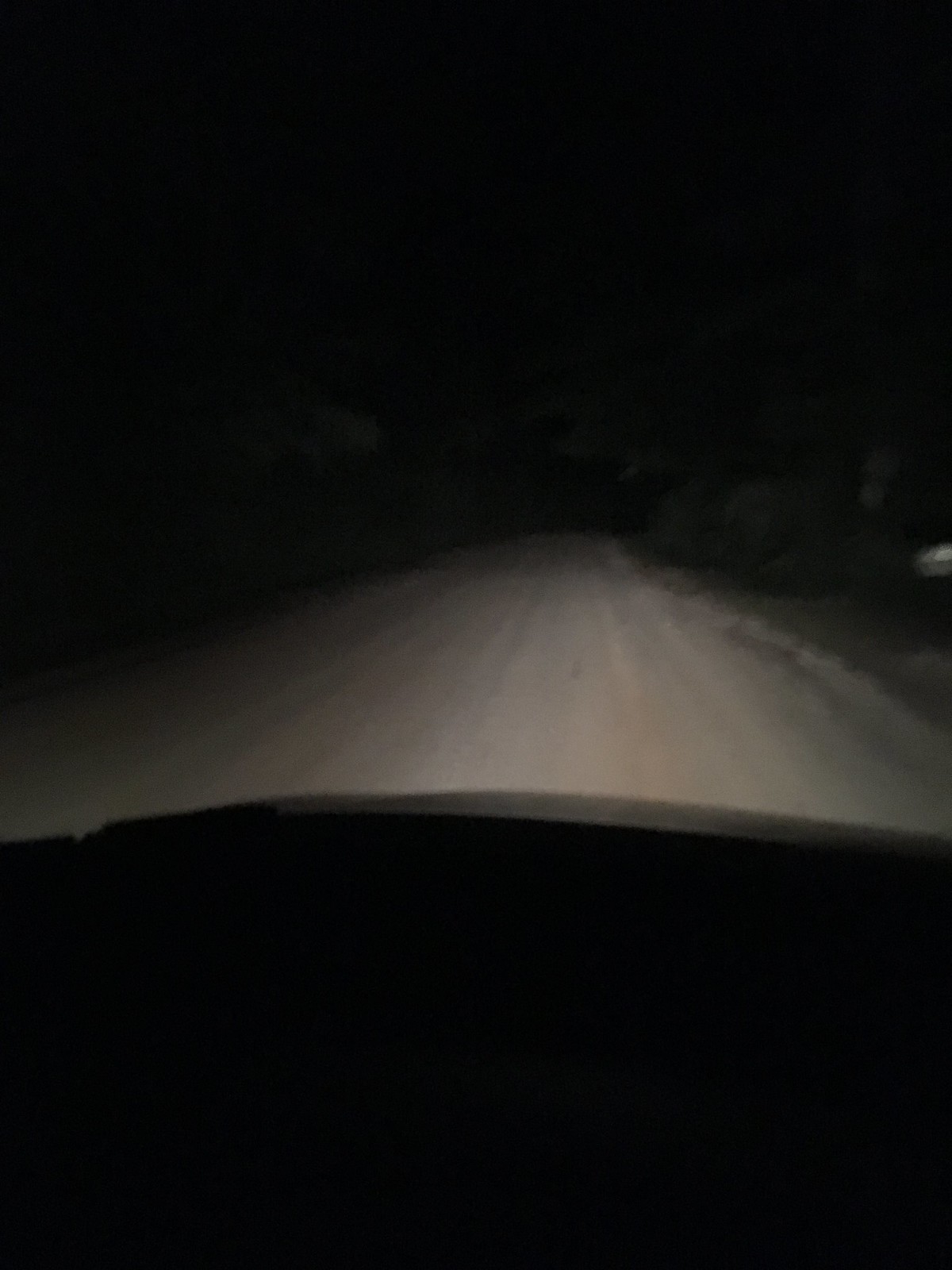The image is notably low-quality, characterized by its dark, blurry, and pixelated appearance. The bottom and upper portions of the image are entirely pitch black, creating a stark contrast with the middle section. In the center, a faint white object or path extends towards the background, though its exact nature is indistinguishable due to the blurriness and poor resolution. To the right of this white path, there is an indistinct object that is also too blurry to identify clearly. This overall lack of clarity and detail makes it challenging to pinpoint specific elements within the scene.